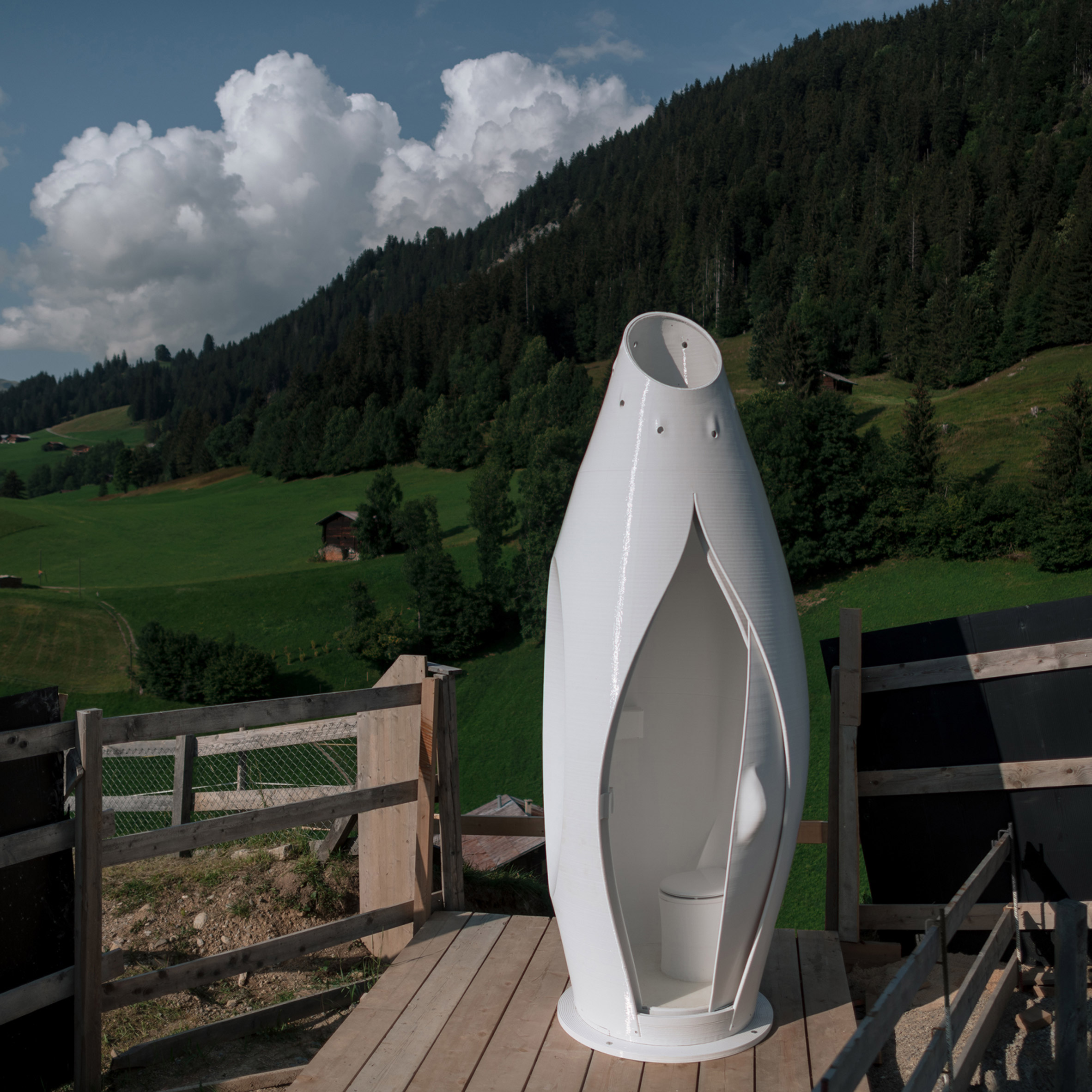The image captures a picturesque farm scene situated on rolling green hills with various dark green trees scattered across the countryside. Prominently, a wooden deck supports a peculiar, futuristic-looking, cylindrical white structure resembling a tulip or a pear-shaped bottle. This smooth, tall object has a flower-shaped doorway with a pointed top and a curved design, giving it an ornamental, space-age aesthetic. The structure functions as a modern outdoor toilet, with its side split open to reveal the interior. To the left and horizontally across the background, a brown fence borders the deck area. In the distance, a tall hill or mountainside rises steeply, adding depth and a natural frame to this unique blend of rustic and contemporary elements.